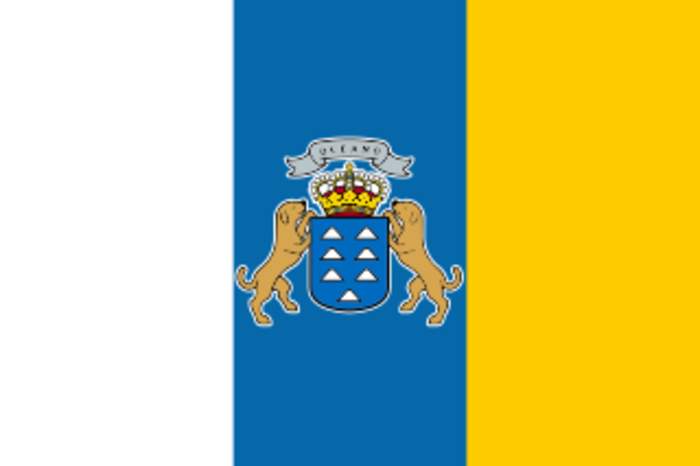The image is a square, split into two halves with a blue left side and a yellowish-orange right side. Dominating the blue half is a detailed crest. The crest features a shield with nine white triangles, held up by two tan dog-like figures standing on their hind legs. On top of the shield sits a red and yellow crown, which appears to be adorned with jewels. Above the crown, a gray ribbon with black, slightly blurry text—possibly stating "Queen"—completes the crest.